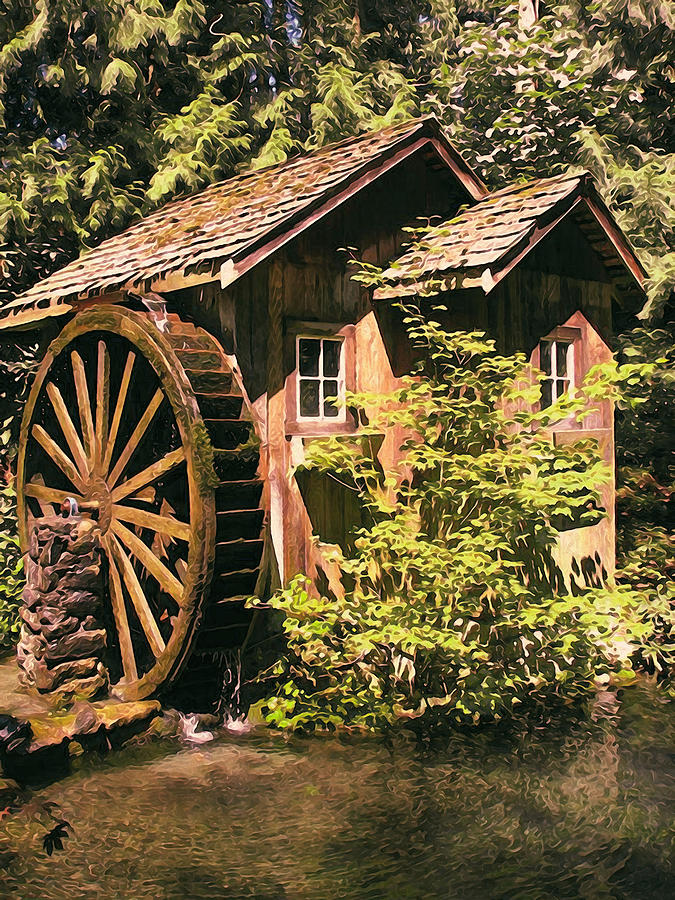This photograph captures a peaceful, bucolic scene of an old wooden sawmill set amidst a lush, green forest. The sawmill, constructed from unpainted timber with a shake or shingle roof, stands serenely at the edge of a murky pond. A large, turning waterwheel, nearly reaching the roofline, dominates the left side of the building. Supported by a stone plinth and integral to the mill's machinery, the waterwheel receives its flow from a gutter along the roofline, spilling water into the wheel and then into the pond below. 

In the foreground, a tall bush extends up to the roof and partially conceals a gabled section, suggesting the presence of a door hidden from view. The mill features white-framed windows with four panes each, adding to its rustic charm. Bright sunlight bathes the scene, highlighting both the natural greenery and the weathered texture of the mill, creating a tranquil and inviting atmosphere—an ideal spot for admiring the serene motion of the waterwheel.